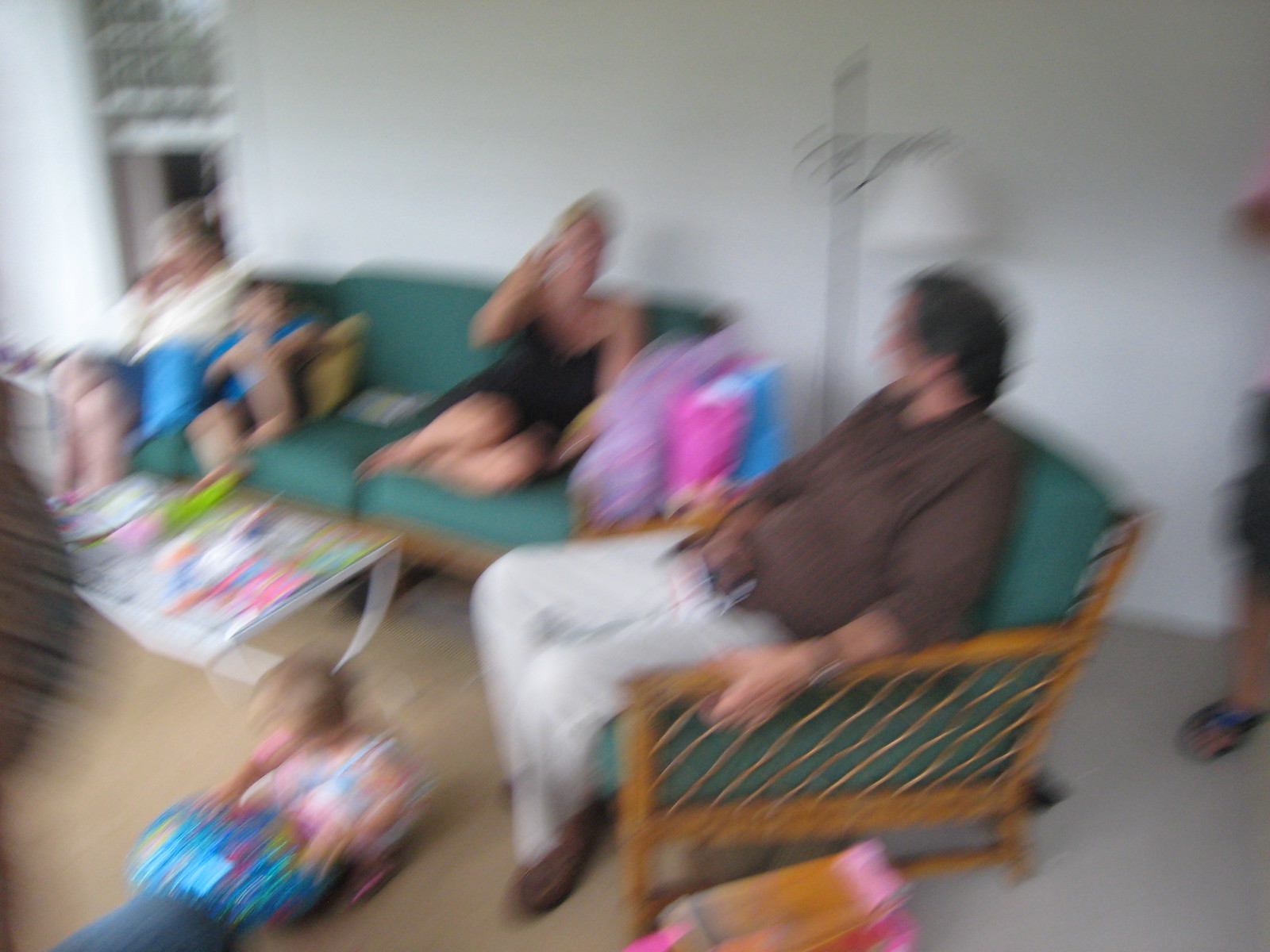This blurry indoor photo captures a lively family scene in a living room. Dominating the upper left corner is a window, positioned above a green couch on which two adults and a child sit. The lady on the edge of the couch has her knees bent and feet up, wearing a black spaghetti-strap dress. Next to her, a child is almost in the center, resting against another person wearing a white shirt and blue pants. Scattered papers, books, and assorted items cover the table in front of the couch. To the right stands a tall lamp, about human height, situated behind a green wicker chair with a man seated in it. The man, with dark hair and a beard, wearing a long brown shirt, khaki pants, and dark brown shoes, engages in conversation with the couch occupants. A toddler, adorned in a dress, plays on the floor in front of him with some toys, while a part of another person's leg and a flip-flop are visible behind the chair.